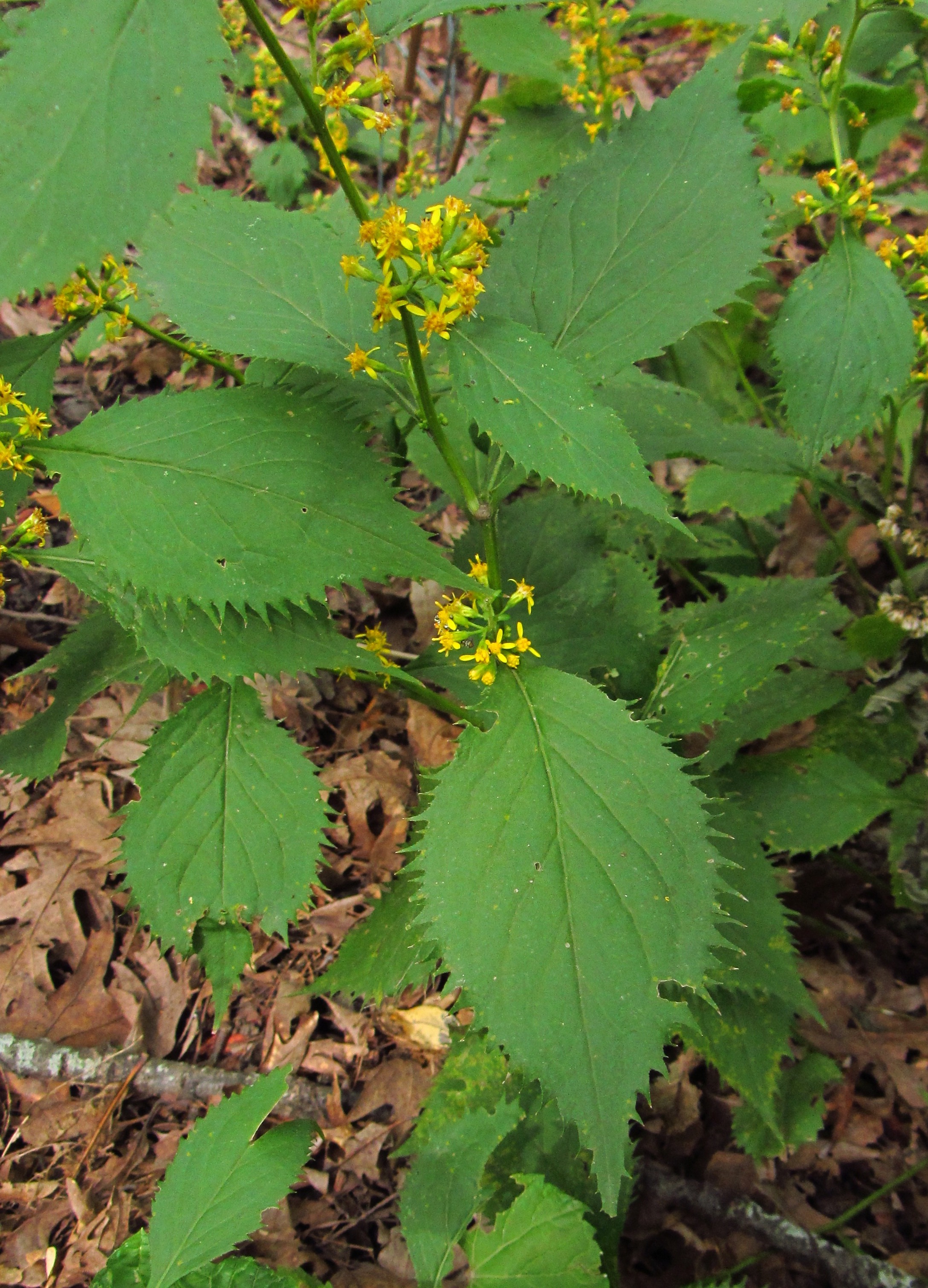The photograph, in portrait orientation, captures an extreme close-up of a dark green plant with pointed, teardrop-shaped leaves that have jagged, serrated edges. The plant is vibrant with clusters of small, three-petaled yellow flowers, resembling miniature daisies, prominently spread along the main stem and throughout its foliage. Surrounding the green plant are numerous brown dead leaves and several large gray twigs, including one notably large twig laying horizontally at the bottom of the image. The plant dominates the composition, filling the frame from top to bottom and left to right, against a wooded background with additional greenery and white flowers mildly visible on the right edge. The photograph represents realism with its detailed depiction of the plant and its surroundings.